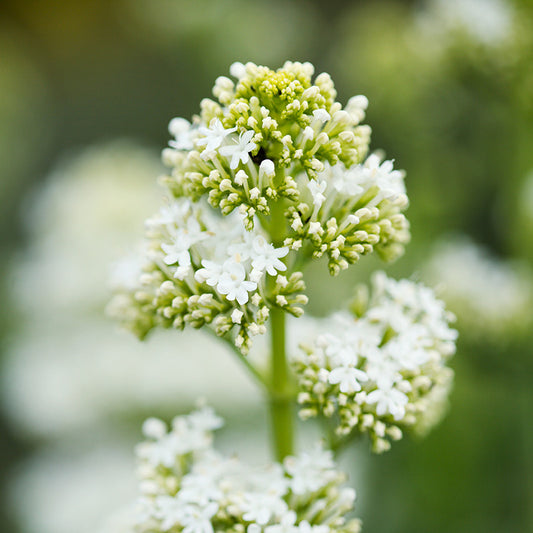This is a square, 4-inch by 4-inch outdoor daytime photograph that draws focus to the center, highlighting a clear depiction of small white-petaled flowers. Each tiny flower, approximately a quarter of an inch in size, features five to six petals with delicate white stamens protruding. These flowers are clustered at the ends of a green stem that rises from the bottom of the image and branches off to the left and right. While the stem and clusters towards the base, as well as the background, are artistically blurred, the focal point remains on the central flowers. The clusters exhibit a mix of fully open white blooms and closed buds tinged greenish-yellow, creating a delicate contrast against the soft, out-of-focus backdrop of additional flowers and foliage.